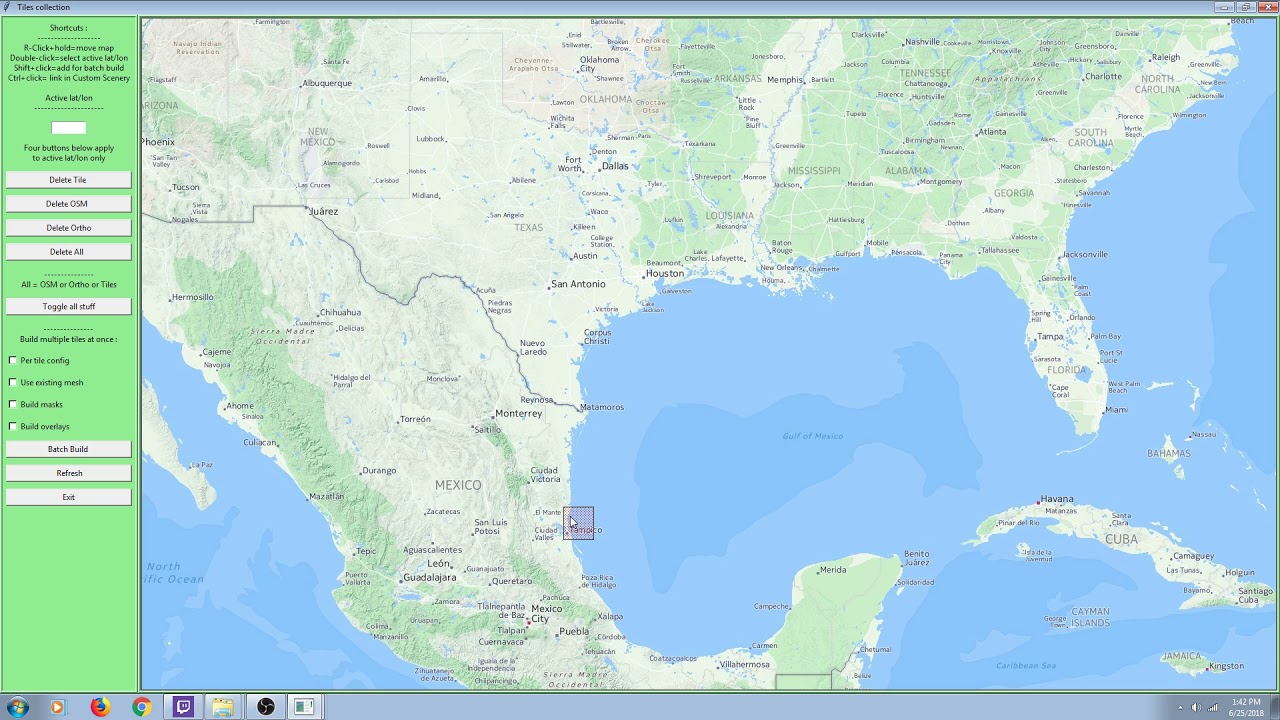A detailed map of the southern and central regions of the United States extends into part of Mexico. At the top, a header with a 3D appearance features a gradient from dark blue at its peak, transitioning through light blue, and ending with shades of light green at the bottom. On the left side, "Tiles Collection" is written in a small, black font next to a blue pen icon.

Beneath this, a long rectangular area with a light green background contains black text in a digital style font. It reads:

**Shortcuts:**

- **R-Click + Hold = Move Map**
- **Double-Click = Select Active Lat/Lon**
- **Shift + Click = Add for Batch Build**
- **CTRL + Click = Link in Custom Scenery**
  
After these instructions, the text clarifies the use of "Active Lat/Lon" for latitude and longitude with a subsequent divider made of dashed lines.

Following this is a small rectangular field with a white background, which appears to be editable due to its 3D effect that gives its border depth. Below this field, again in small, black digital font, it states: "Four buttons below apply to active lat/lon only."